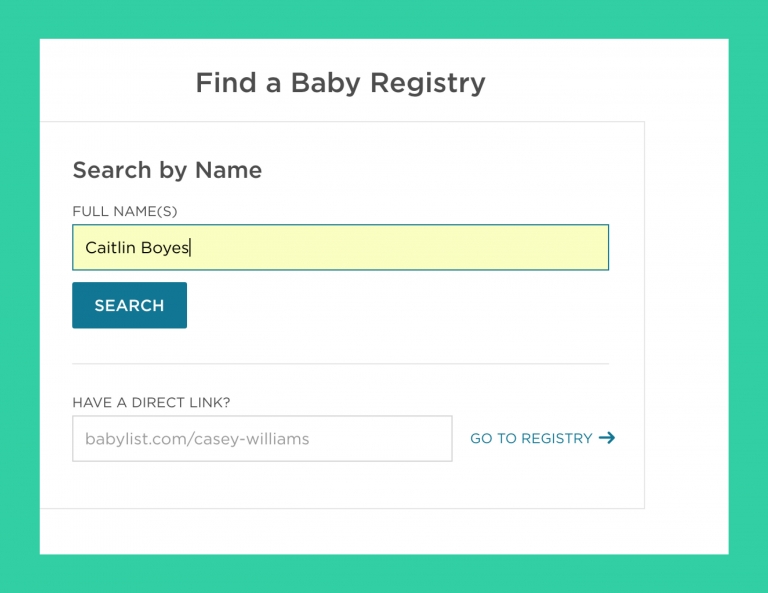The image showcases the "Find Baby Registry" section of a website, which provides a search engine to locate a baby registry. The interface is neatly designed with a distinct layout. A green square border frames the entire section, drawing attention to the content within.

At the center lies another square with a clean, white background. At the top of this square is the heading "Find a Baby Registry," indicating the purpose of the section. Below this, on the left side, there is the option to "Search by Name."

Under this heading, the term "Full Names" appears, suggesting that users should input full names for accurate search results. Adjacent to this label is a text input box where users can type the name they wish to search for. Currently, the name "Caitlin Boyes" is entered in this box, clearly spelled out as C-A-I-T-L-I-N B-O-Y-E-S.

Beneath the name input field, there is a prominent blue button with white text that reads "Search," inviting users to initiate their search. A subtle line separates this section from the following part of the interface.

Next, there's a prompt asking "Have a direct link?" with further details. Below this question, there is a URL displayed as "babylist.com/casey-williams." To the right of this URL, there is a "Go to Registry" button accompanied by a right-pointing arrow, suggesting navigation to the specified registry. This thoughtfully organized design aims to provide a clear and user-friendly experience for individuals searching for a baby registry.